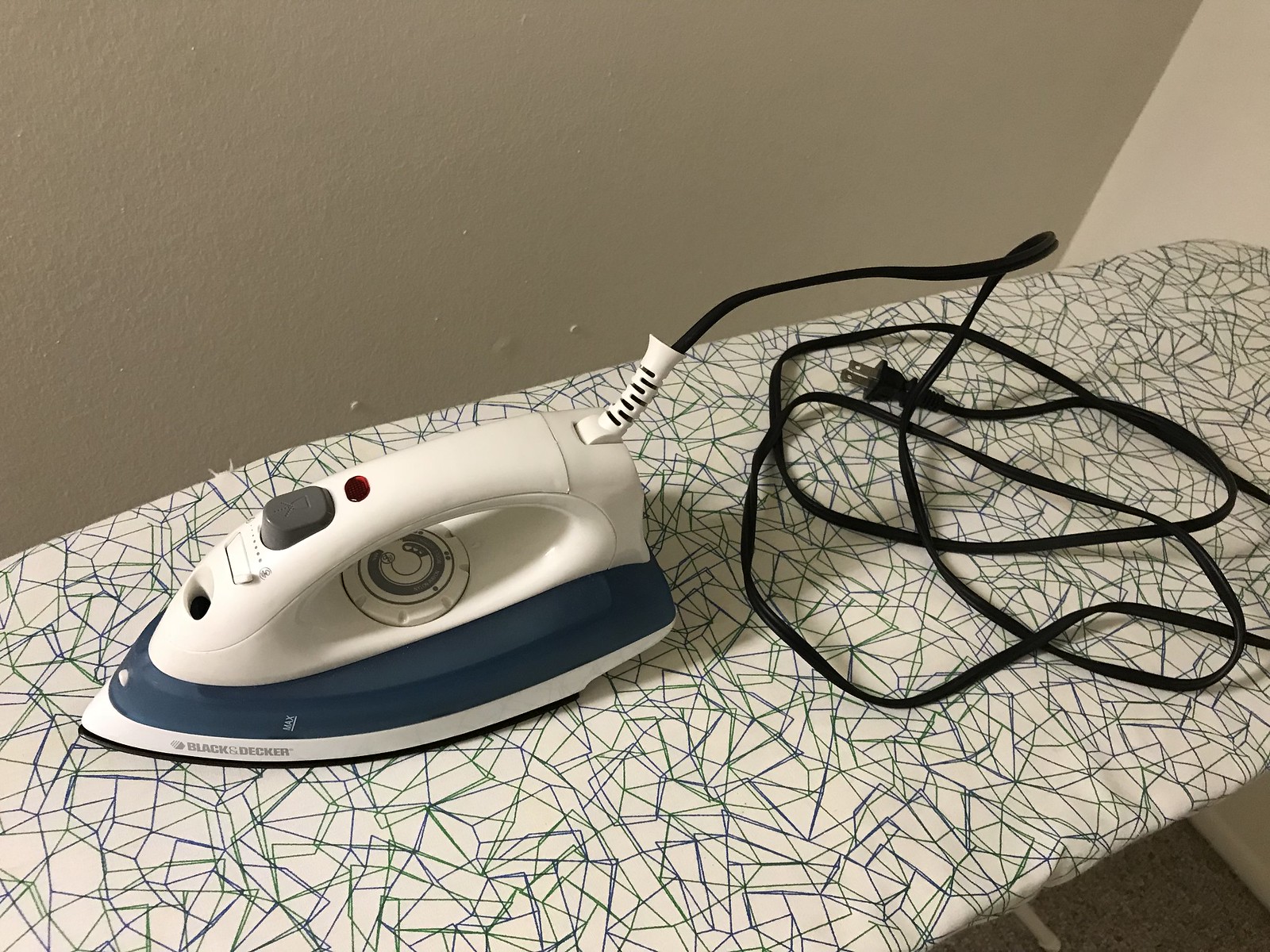This color photograph features a detailed close-up of an iron resting on an ironing board. The ironing board, partially cut off in the image, has a white surface adorned with squiggly lines of black, green, and blue, and stands on white legs. The iron, situated towards the left of the picture with its tip pointing to the bottom left, boasts a two-tone design. Its body is primarily off-white cream, accentuated with a navy blue band near the bottom, where "Max" is written, and another off-white band at the very base displaying the brand name "Black & Decker" in gray text.

The iron’s faceplate lies flat against the ironing board, indicating it is safely switched off. A large grey button and a red indicator light are on the neck of the iron, with a circular dial positioned beneath the handle. A black, flexible electrical cord extends from the top back of the iron, coiled neatly to the right and ending in a two-pin plug resting on the ironing board.

The background features a light pink or magnolia wall running horizontally across and then turning at a 90-degree angle towards the camera. Additionally, a patch of gray carpet is visible in the bottom right corner of the image.